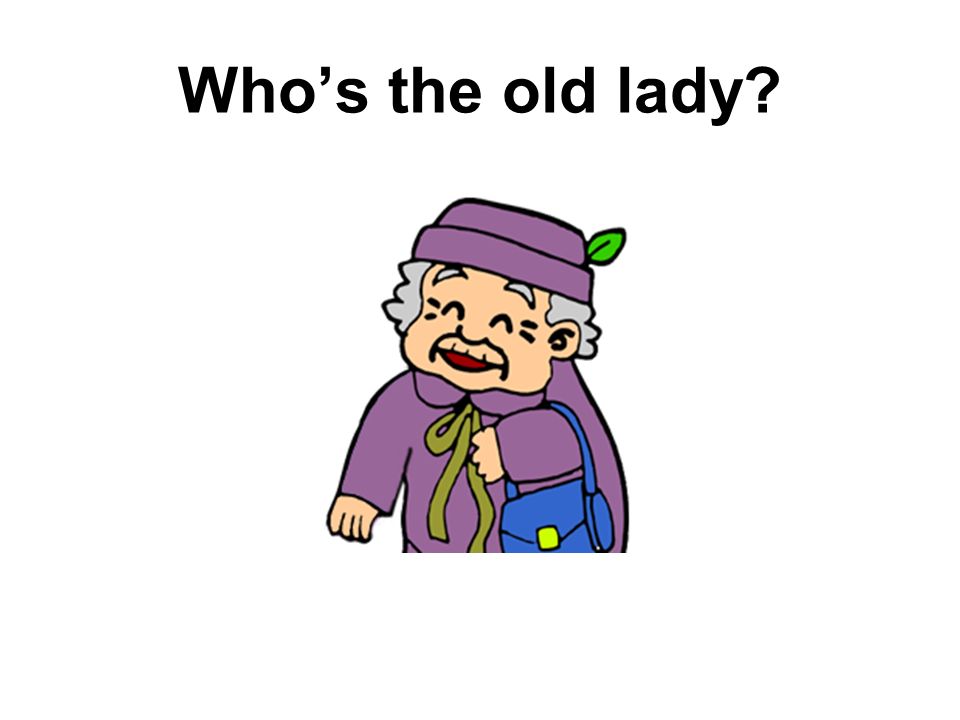This image features a cartoon illustration of an elderly woman centered against a white background. She is depicted wearing a purple hat adorned with a small green leaf on the right side, and her short gray hair peeks out from beneath it. Her matching purple coat, complemented by a possible green scarf or decorative tie, covers her as she smiles gently with red lips and shut eyes, showcasing wrinkles beside them. In her left hand, she holds a blue purse with a lime green clasp. Above her, the black text reads, "Who's the old lady?"